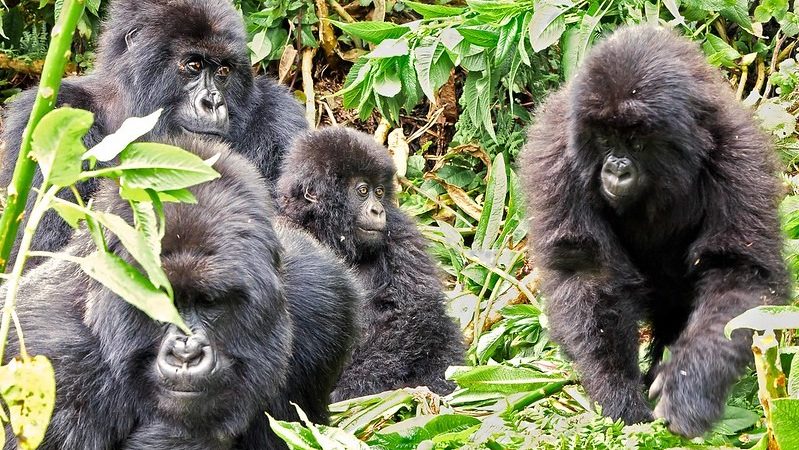This image captures a family of four gorillas amidst lush green foliage with some brown stalks. The three adults and one infant are positioned against a background teeming with green leaves. The largest male gorilla, situated prominently in the lower foreground, gazes intently at the camera, displaying an imposing presence. To his left, an upright tree stalk adorned with vibrant green leaves partially obstructs the view of an adult female gorilla seated behind, who is looking off to the right in the same direction as the infant. The young gorilla sits in the lap of the female, their shared focus turned to the right. On the right side of the image, an adolescent gorilla stands independently on all fours, looking downward. The textured black hair of each gorilla contrasts vividly with the surrounding greenery, adding depth to this captivating portrayal of gorilla life in their natural habitat.